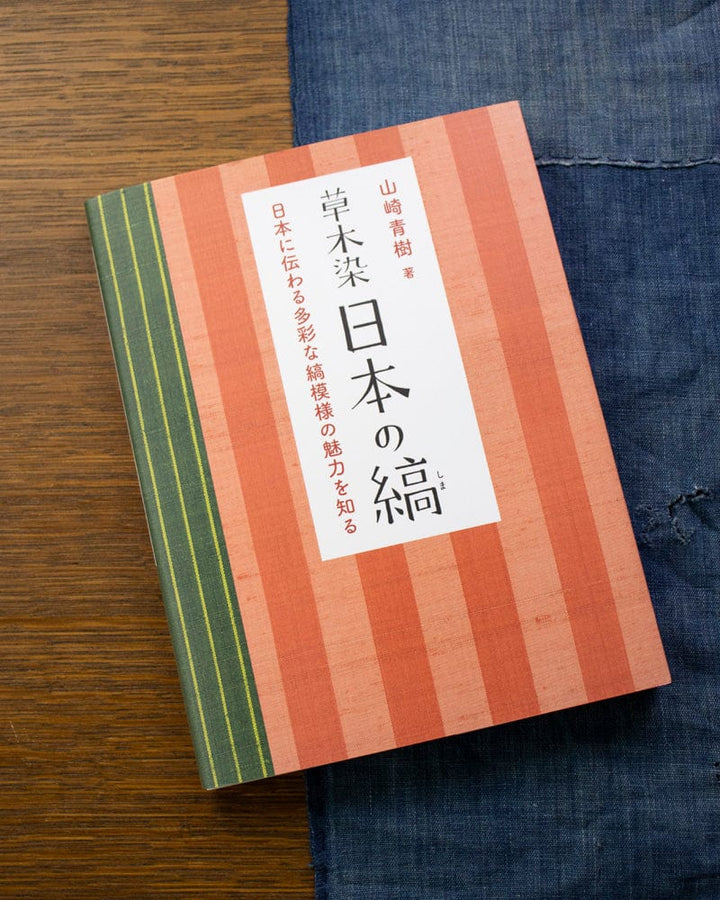The image portrays a small book, resembling a diary or journal, showcasing Japanese plant-dyed stripe patterns. The book features vertical stripes in various shades of orange, including darker and lighter hues, as well as a binding in green with lighter goldish-green stripes. The cover is adorned with Japanese text detailing the book's title and description. This book is placed on a denim fabric, likely part of a pair of jeans with a visible rip or hole, suggesting a potential connection to sewing or pattern design. The entire setup rests on a wooden surface with visible horizontal grain.